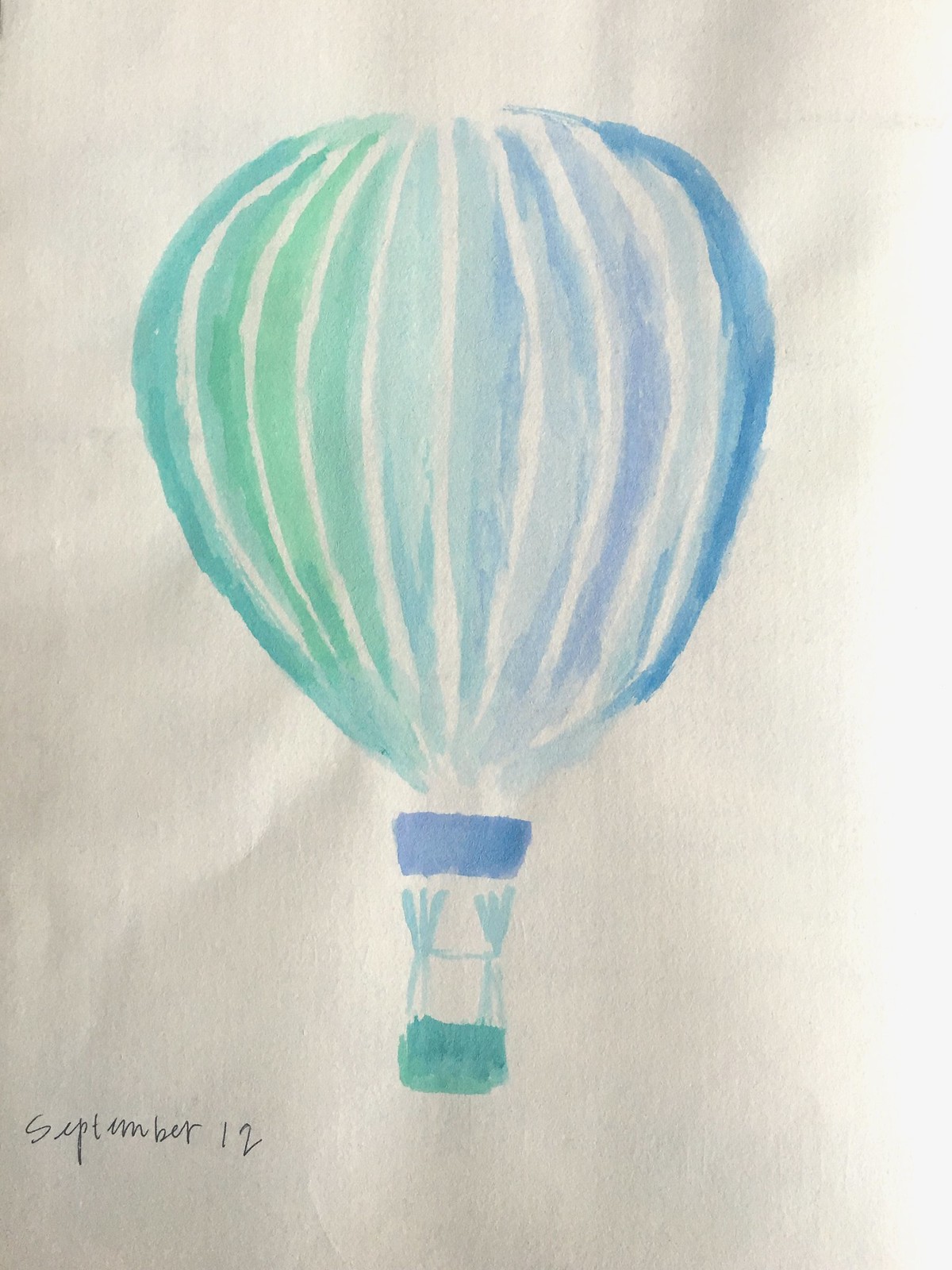This watercolor sketch captures the whimsical essence of a hot air balloon floating in mid-air. The balloon itself is an intriguing blend of light green on the left side, seamlessly transitioning into various shades of blue, from light to dark, as it progresses towards the right. Despite being a rough sketch with minimal detailing, the vibrant colors bring it to life. The basket, painted in a striking teal, complements the overall palette, while a solid blue band at the balloon's base adds a subtle yet cohesive touch. The entire composition is set against the pristine backdrop of a white piece of paper. In the bottom left corner, the date "September 12" is inscribed in elegant black ink, adding a personal and temporal element to the artwork.